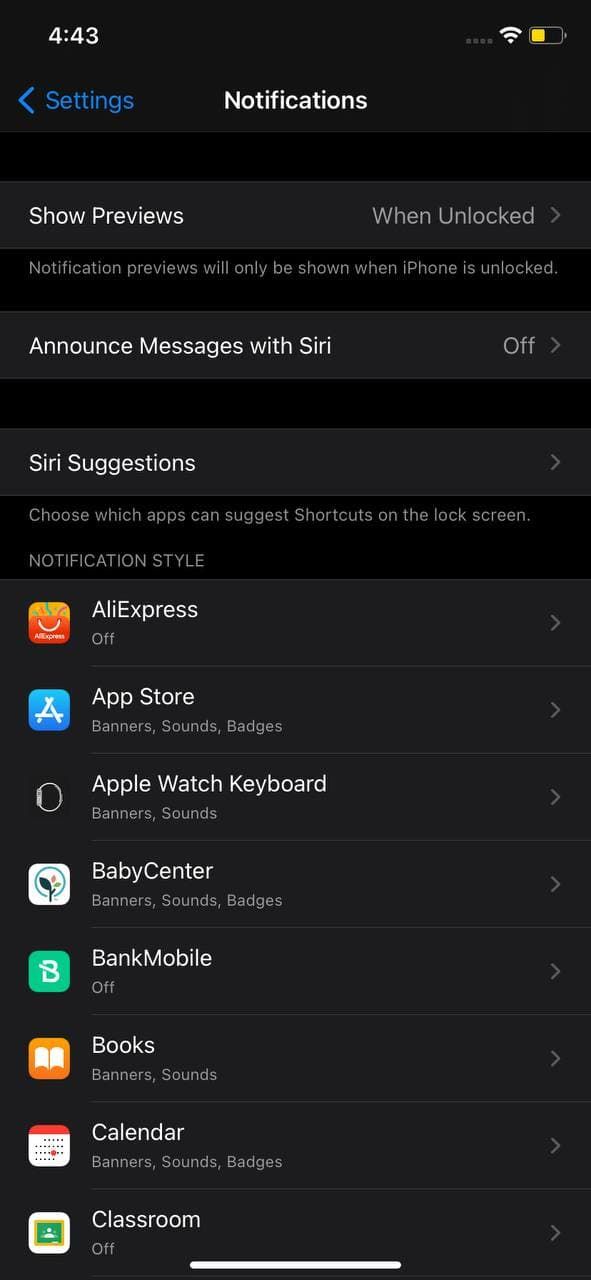**Caption:**

The screenshot displays a phone interface with a black background. At the top of the screen, the time is shown as 4:43, along with icons for signal strength and battery level on the right side. Just below this, a blue back arrow is present, labeled "Settings," with the "Settings" text in blue. In the center of this line, the word “Notifications” appears in white.

Below this header, a section labeled "Show Previews" is visible. On the left, the option is labeled in white, while on the right, a lighter, faded gray text reads "When Unlocked," accompanied by a small right-pointing arrow. Beneath this section, a sentence clarifies: "Notification previews will only be shown when iPhone is unlocked."

The next section, titled in bold white letters, is "Announce Messages with Siri," indicating that this feature is turned off. Below this is another section labeled "Siri Suggestions," featuring a right-pointing arrow. It explains with further text: "Choose which apps can suggest shortcuts on the lock screen."

Finally, the screenshot lists various apps under the "Notifications" section, complete with their icons. The listed apps include AliExpress, App Store, Apple Watch, Keyboard, BabyCenter, Bank Mobile, Books, Calendar, and Classroom.